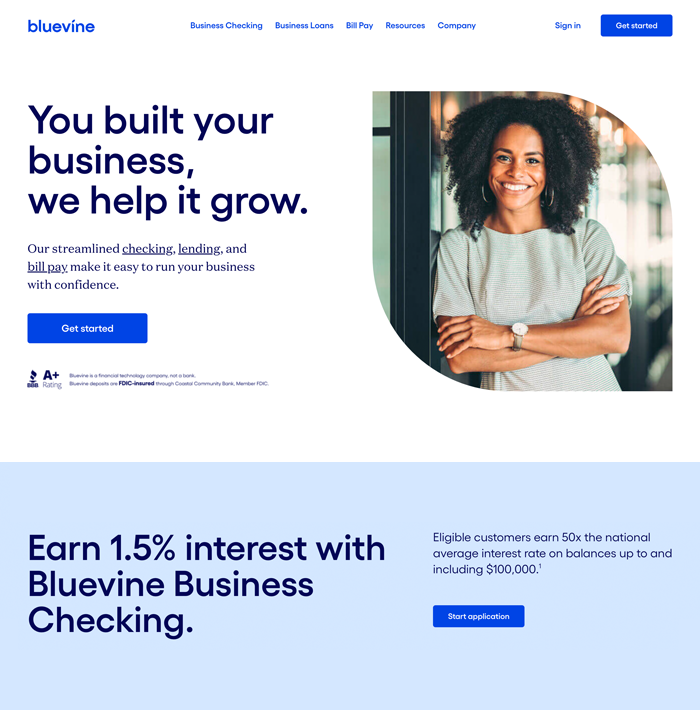This image is a promotional webpage for Blue Vine, prominently featuring their brand and services. In the top left corner, the Blue Vine logo, colored in blue, is clearly visible. To the right of the logo, there is a horizontal navigation menu with five categories: Business Checking, Business Loans, Bill Pay, Resources, and Company. 

On the top right corner, two additional options are presented: 'Sign In' and 'Get Started', with 'Get Started' displayed in white text on a blue rectangular background, making it stand out. 

The central part of the image showcases a diverse female professional with crossed arms, wearing a watch on her left wrist and earrings. She has an Afro hairstyle and a deep skin tone. To her left, a bold message reads, "You built your business, we help it grow." Beneath this slogan, a smaller text details Blue Vine's offerings: "Our streamlined checking, lending, and bill pay make it easy to run your business with confidence." Another 'Get Started' button, also in white text, is positioned below this description.

The bottom section of the image contains two boxed announcements. On the left, it highlights "Earn 1.5% interest with Blue Vine Business Checking." On the right, there's a call to action: "Start Application."